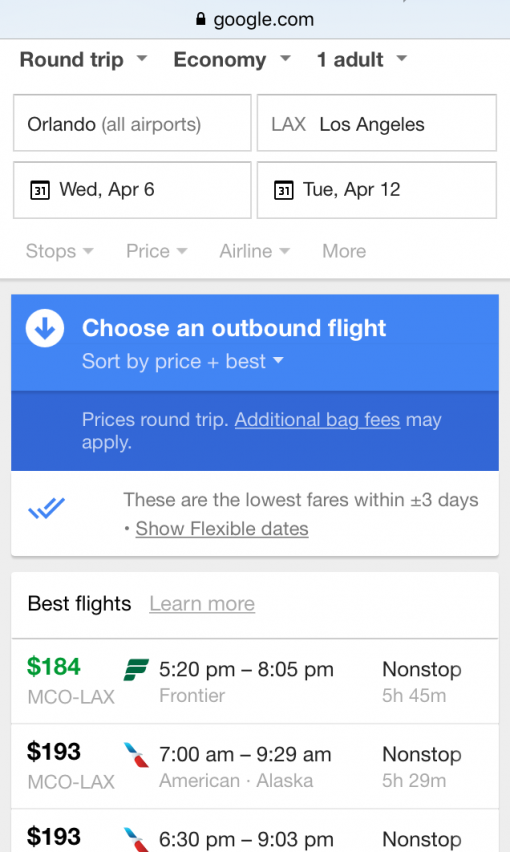The image displays a flight search results page with various elements and details organized in a user-friendly layout. 

**Top Section:**
- **Top Banners:** Grey background with a black padlock icon, indicating a secure connection, and "google.com" below it. This section also includes black text on a white background with options labeled "Round Trip," "Economy," and "One Adult," each accompanied by a downward arrow for further selection.

**Left Sidebar:**
- **Search Inputs:** A grey box on the left contains the departure location "Orlando, All Airports" (abbreviated as 'MCO'), and the destination "LAX, Los Angeles." Below, there are calendar icons highlighting the travel dates: "Wednesday, April 6th" and "Tuesday, April 12th."

**Filter Section:**
- **Grey Box Filters:** Options to filter by "Stops," "Price," "Airline," and "More," each with a downward arrow to refine the search results further.
  
**Main Results Area:**
- **Sort Options:** A grey outlined box contains controls to "Choose an airport flight," "Sort by price," with additional sorting options indicated by text such as "Best" and a downward arrow. There is also a white circle and a grey arrow-down icon for additional sorting options.
  
- **Price Notice:**
   - A dark blue background banner with white text indicates that prices are for round-trip flights and additional bag fees may apply. A double blue check mark accompanies the text "These are the lowest fares within ±3 days," with an underlined option "Show flexible dates."

- **Flight Options:**
  - **First Option:** 
    - Price: $184
    - Route: MCO-LAX
    - Departure: 5:20 PM, Arrival: 8:05 PM
    - Airline: Frontier
    - Duration: 5 hours 45 minutes
    - Additional Info: Non-stop flight.
  - **Second Option:** 
    - Price: $193
    - Route: MCO-LAX
    - Departure: 7:00 AM, Arrival: 9:29 AM
    - Airline: Likely American Airlines or Alaska
    - Duration: 5 hours 29 minutes
    - Additional Info: Non-stop flight.
  - **Third Option:**
    - Price: $193
    - Route: MCO-LAX
    - Departure: 6:30 PM, Arrival: 9:03 PM
    - Airline: Likely American Airlines or Alaska
    - Additional Info: Non-stop flight.

**Footer Section:**
- **Best Flights:** A white square with black text marked "Best Flights" and grey font underlined "Learn More." 

The overall layout of the page is designed for ease of use, highlighting major travel details, fare options, and filtering mechanisms to help users quickly find suitable flight options.